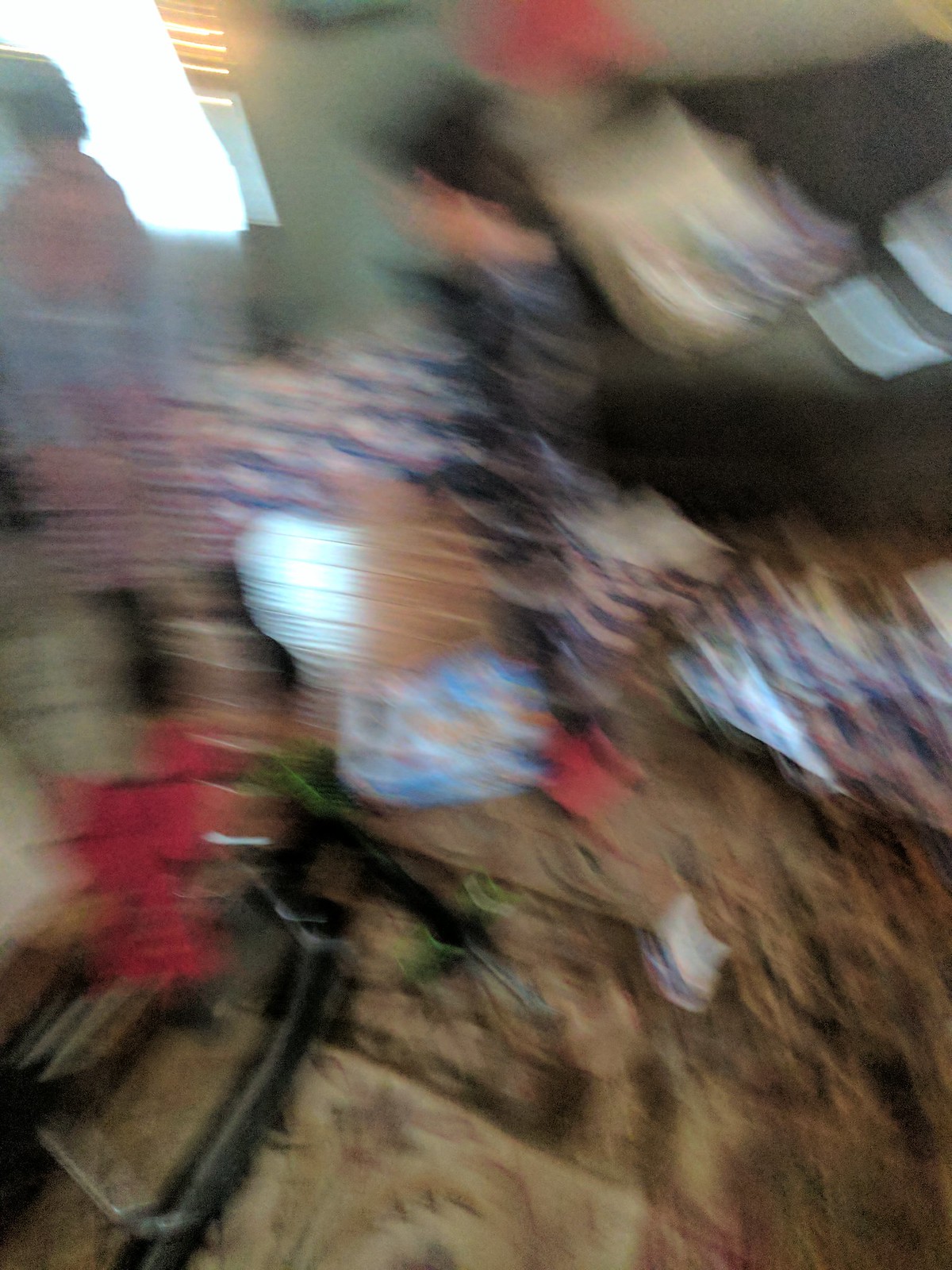In this very blurry and out-of-focus photograph taken inside a building, several indistinct shapes fill the frame. At the bottom of the image, there's what seems to be an area rug with a pattern of black, brown, and cream colors. In the lower left-hand corner, a black object constructed of cylindrical segments is visible. Directly above the object, there is a red blurry shape, which might be flowers. Across the center, a series of blurred shapes are dominated by wavy horizontal lines in peach, black, and brown. To the upper left-hand corner, a square of light suggests a window, next to which stands a figure dressed in an orange shirt, likely with short, dark hair, facing away from the camera. There is also a possible view of a table surface with a light brown placemat, scattered with floral designs, and what may be a stack of white dishes and a hand near them. Overall, the image is obscured, making the details difficult to discern, but these elements emerge through the blurriness.